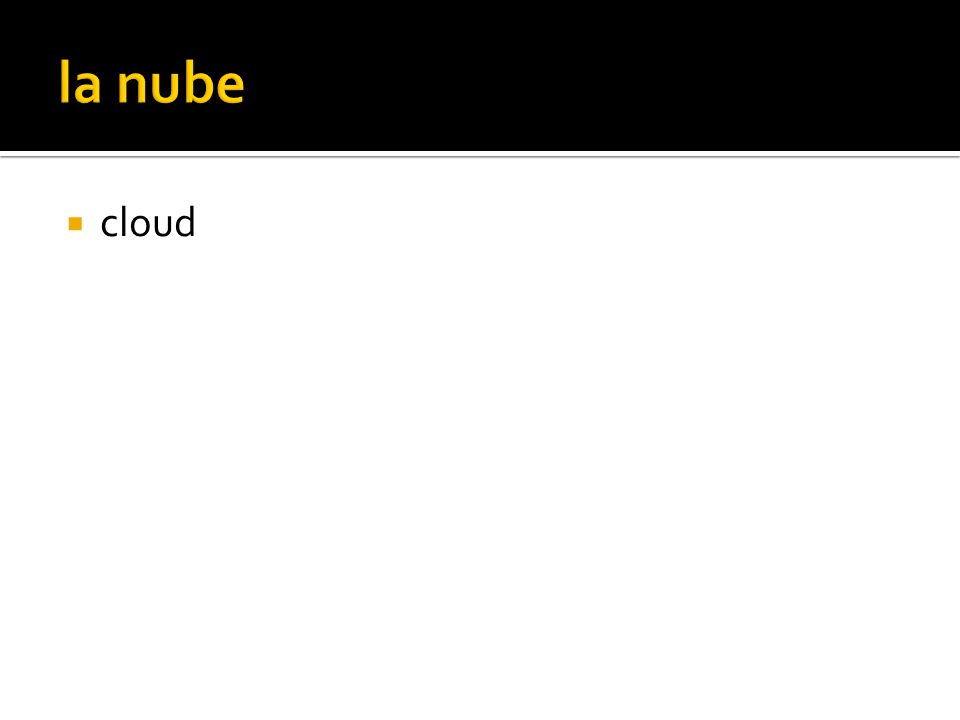This image presents a minimalistic design with a focus on textual elements. At the top, there is a solid black rectangle extending horizontally, within which, towards the left side, the word "lanube" is displayed in all lowercase, yellow Arial-like font. Directly beneath this rectangle runs a thin black line. Below this line, there is a yellow square bullet point followed by the word "cloud," written in lowercase black Arial-like font. The entire background underneath the black rectangle and thin line is stark white, giving the image a clean, uncluttered appearance reminiscent of a simplistic PowerPoint slide.